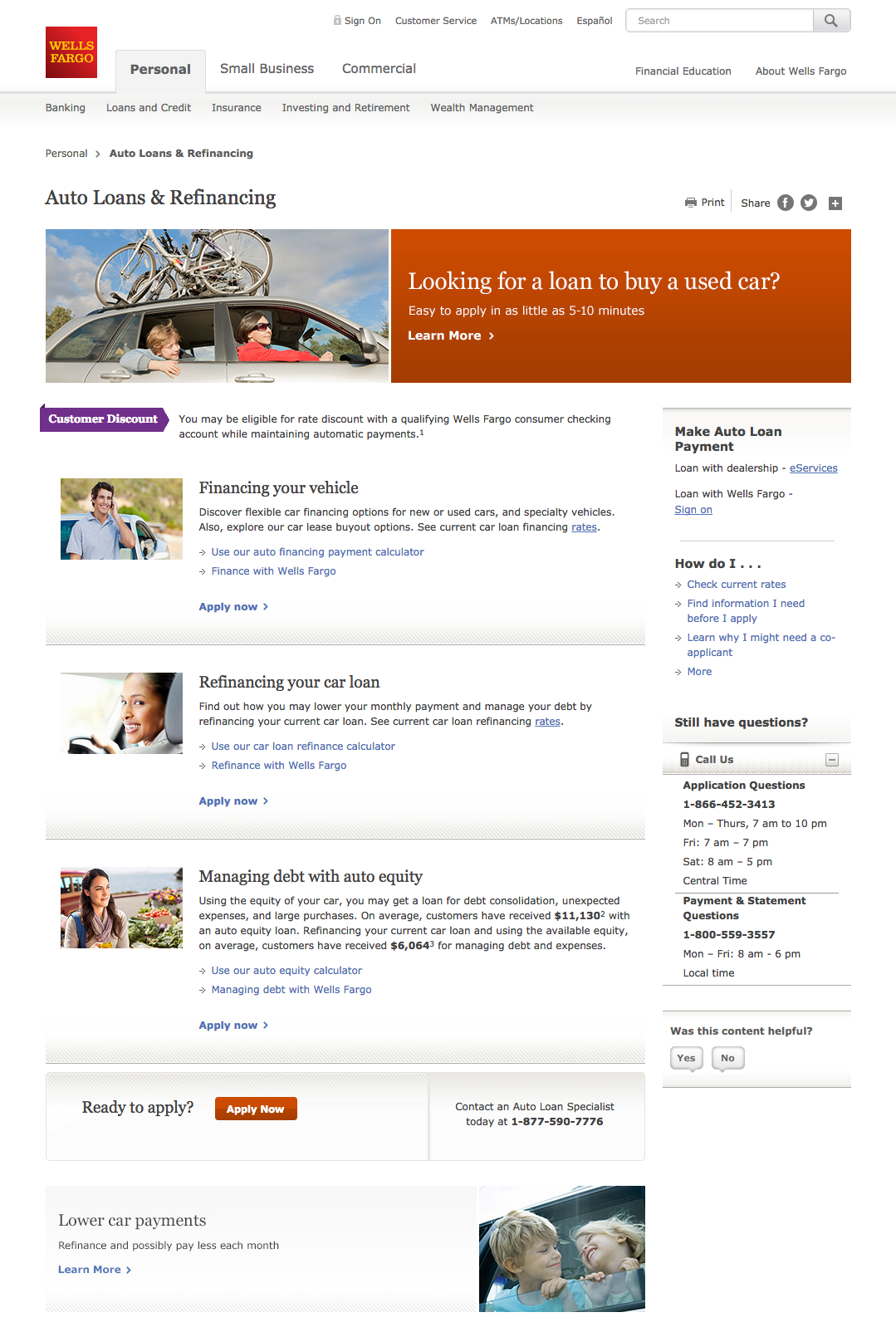This is a detailed screenshot of the Wells Fargo web page, characterized by a predominantly white background with red accents and black text, while the hyperlinks appear in blue. The top of the page features a white header, prominently displaying the Wells Fargo logo in the upper left corner. Adjacent to the logo on the right is a navigation menu with tabs for "Personal," "Small Business," and "Commercial" services.

Beneath this header is the main content of the page, beginning with an expansive banner titled "Auto Loans and Refinancing." The left side of the banner showcases an engaging image of a family standing beside a car, evoking a sense of security and satisfaction. On the right side of the banner, there is a prominent red rectangle highlighting an option for securing a loan to buy a used car, accompanied by a line of text that is not fully legible. This section also includes a "Learn More" link for additional information.

Further down, the page is organized into a series of informative rectangles, each containing images and pertinent details about various services. A sidebar runs along the side, hosting a collection of useful links for easy navigation.